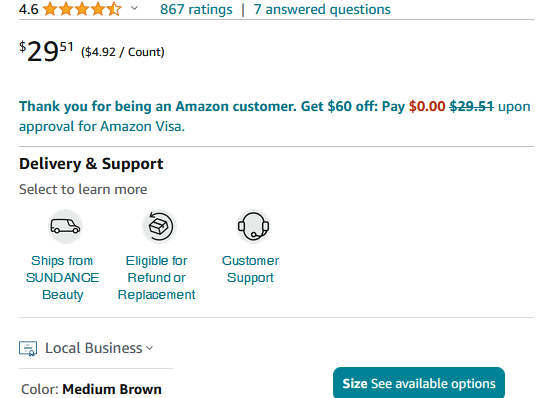This screenshot displays a product review interface on Amazon. The review section highlights a product with a 4.6-star rating based on 867 reviews, accompanied by seven answered questions, all of which are hyperlinked in blue. The product price is listed as $29.51. A promotional message underneath thanks customers for shopping on Amazon and offers a $60 discount, with the possibility of paying $0 upon approval for an Amazon Visa, also highlighted in blue.

Following the promotional content, there's a section labeled "Delivery and Support", prompting users to "Select to learn more". It mentions that the item ships from Sundance Beauty and is eligible for refund or replacement, as well as customer service support. A gray demarcation line follows.

Below this line, there's a segment dedicated to "Local Businesses", detailing the product specifics: the color is identified as medium brown, the size is noted as C, and there are additional options available through a clickable blue tab.